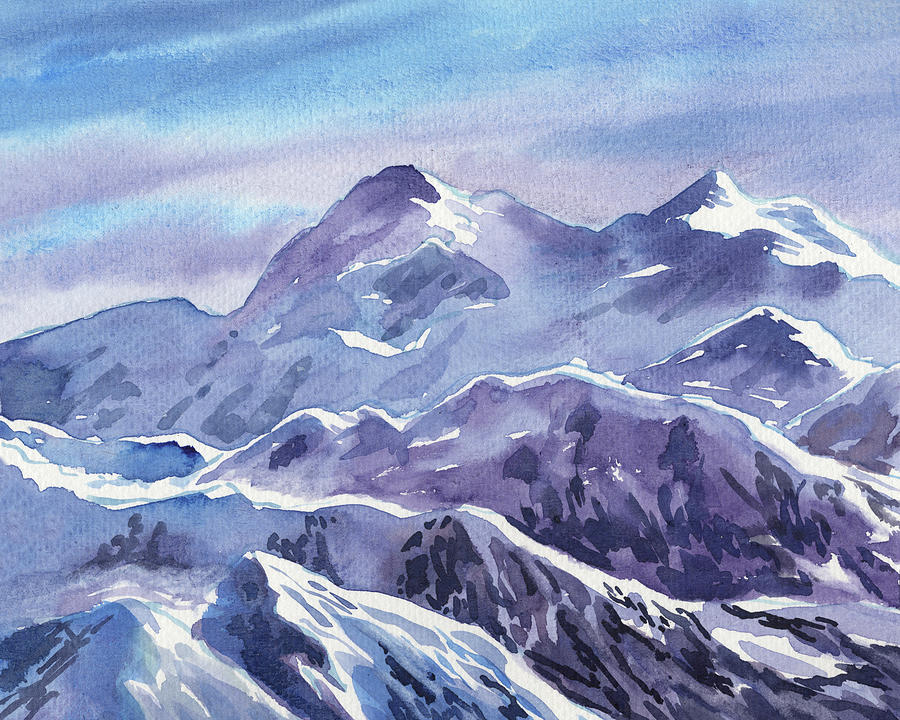This watercolor painting depicts a majestic mountainous landscape with snowy peaks bathed in different shades of blue, purple, and white. The sparse scene is devoid of trees, emphasizing the rugged, barren rock formations. The image captures a clear, sunny day, with light and shadow contrasting beautifully; light illuminates the right side while shadows stretch across the left. The sky consists of a gradient of hues, transitioning from light blues and purples to darker shades towards the top. The overall atmosphere is serene and ethereal, making the painting both visually compelling and believable.